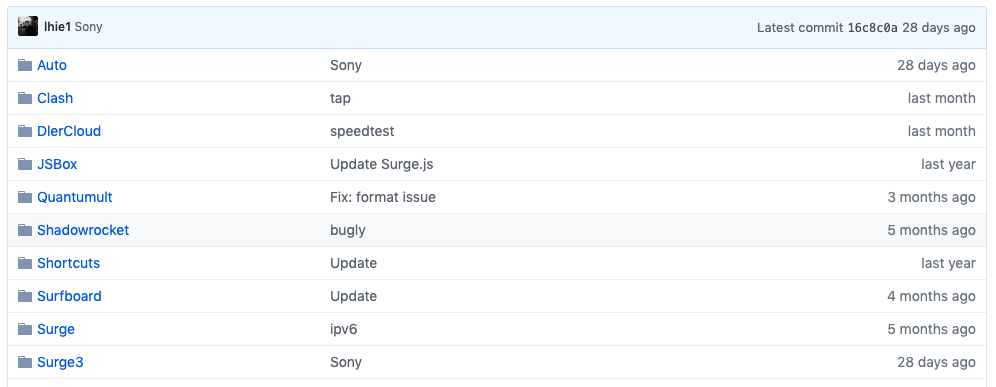The image depicts a section of a software repository interface labeled "LHIE1Sony." At the top, there's a light blue band stretching from left to right. On the top-right corner, the text reads, "Latest Commit COMMIT 16CBC0A 28 Days Ago." Below this is a column on the left listing various files: auto, clash, direcloud, jsvbox, quantumult, shadowrocket, shortcuts, surfboard, surge, and surge 3, each with a corresponding file icon.

In the middle section, there are a series of terms without explicit context: Sony, taps, tests, speed test, update, surge.js, fix: format issue, bulgly, update IPV6, and Sony. 

On the right side, there are timestamps displayed for each entry: "28 days ago," "last month," "last month," "last year," "three months ago," "five months ago," "last year," "four months ago," "five months ago," and "28 days ago." Notably, the entry for "shadowrocket" is highlighted with a gray background, distinguishing it from the others which have a white background.